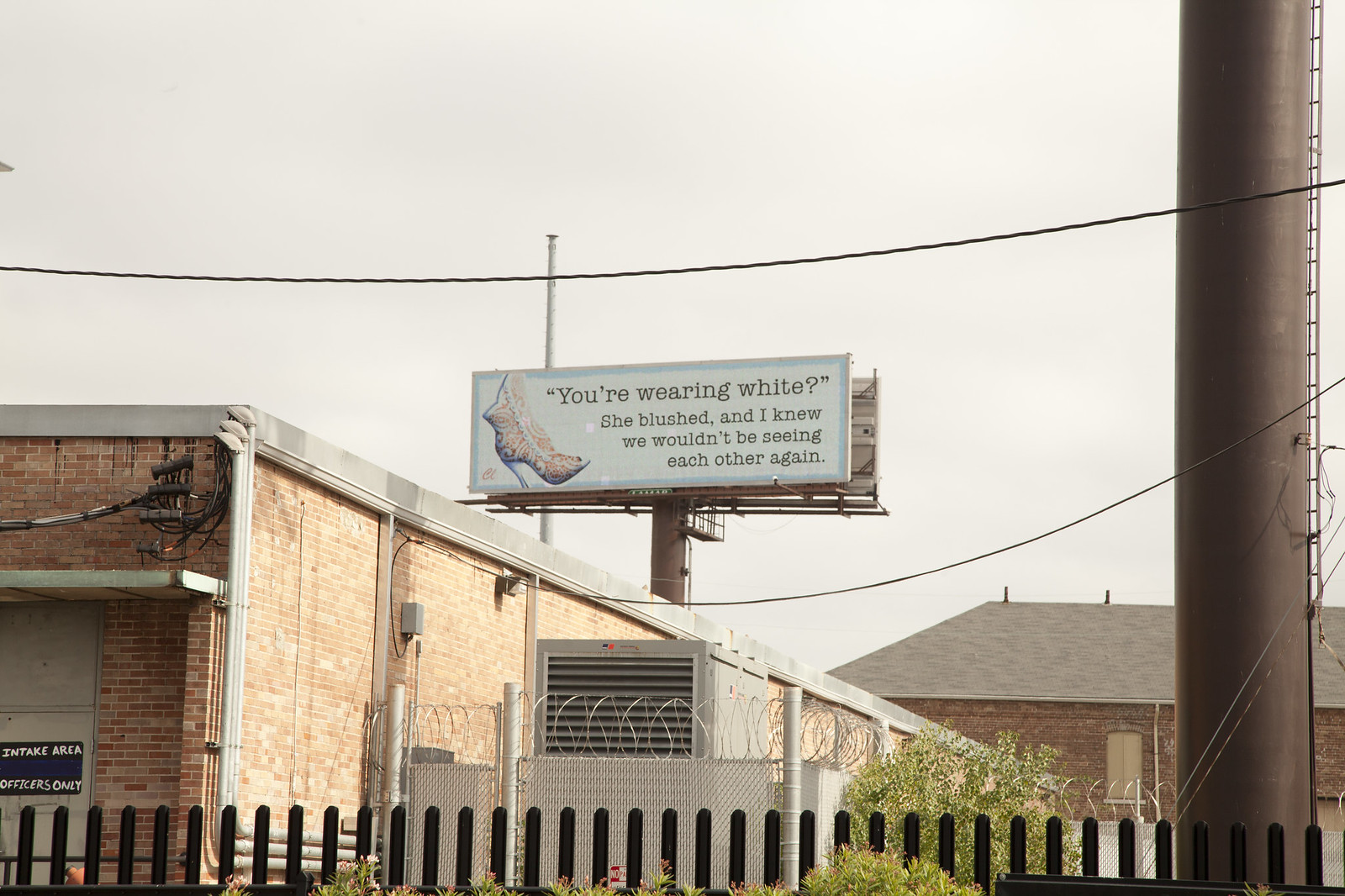The image captures an industrial scene featuring what appears to be a high-security facility, possibly a jail or police station, surrounded by a barbed-wire topped, chain-linked fence. In the foreground to the left is an industrial building with a designated intake area for officers only, emphasizing the security nature of the location. Prominently visible is a thick, brown smokestack-like pole with a ladder attached. Suspended power lines droop across the frame, bisecting the overcast sky. Behind this setting, a billboard with a white background advertising a high-heeled ankle boot features a woman's foot. The billboard text, in brown writing, reads: "You're wearing white. She blushed and I knew we wouldn't be seeing each other again." The billboard and its contents stand out amidst the scene, adding a peculiar juxtaposition to the otherwise stark and secured environment.